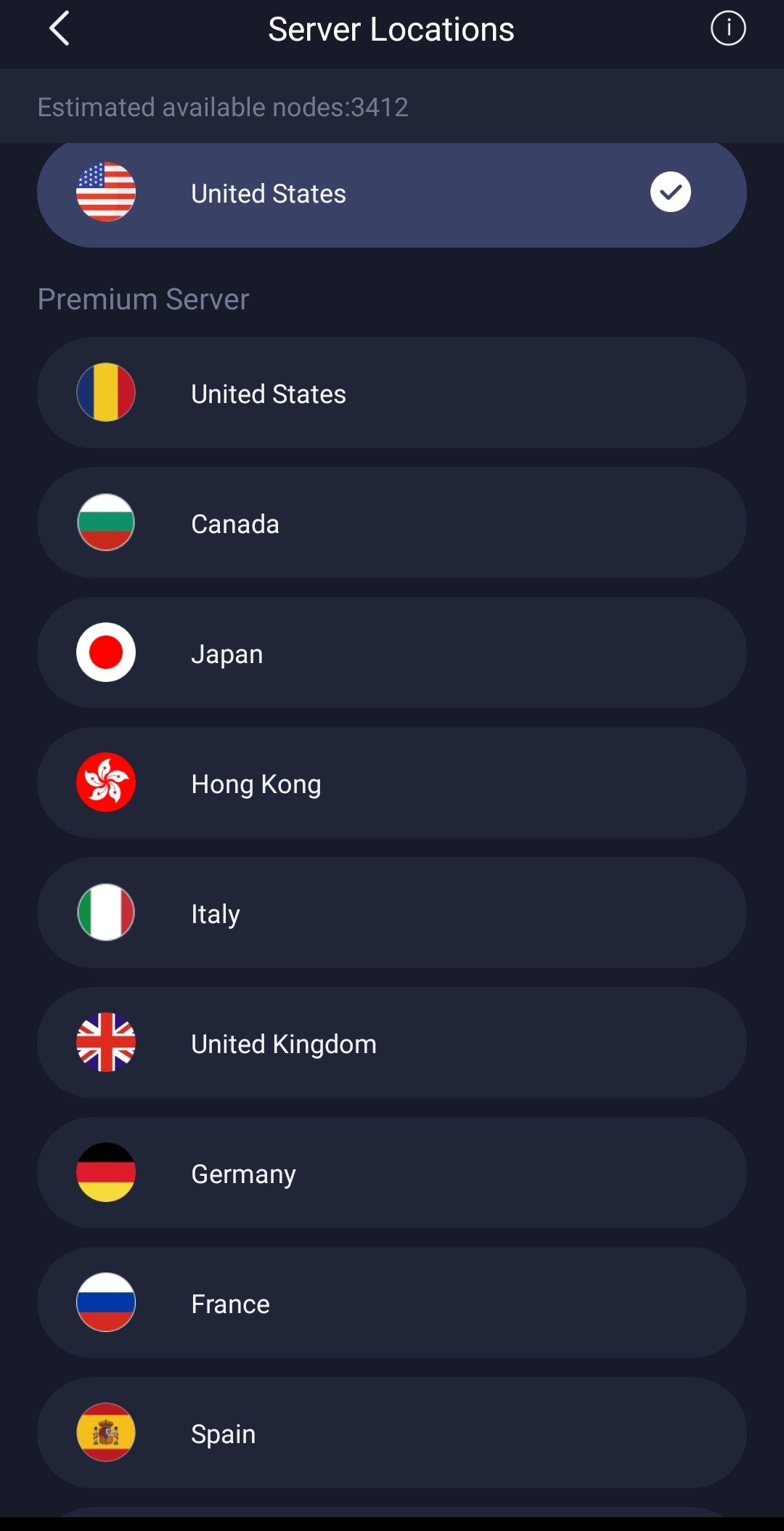The image depicts a smartphone screenshot showcasing a virtual private network (VPN) server selection interface. The background features a dark blue-black hue with white text prominently displayed for readability. At the top of the screen, there are navigation icons: a back button situated on the left and an information button on the right.

The section titled "Server Locations" lists multiple countries where VPN servers are available, outlined in light blue ovals to distinguish them from the background. Each country is accompanied by its national flag for easy identification. Below the "Estimated Available Nodes" label, which indicates 3,412 potential nodes, the United States is checked as the selected server, marked as a premium option.

Besides the United States (marked with an incorrect flag), other countries listed include:

- Mexico
- Canada (also shown with an incorrect flag)
- Japan
- Hong Kong
- Italy
- United Kingdom
- Germany
- France
- Spain

Despite the correct inclusion of Germany's flag, there are noticeable errors in the flags for Canada and the United States, with Canada depicted using Portugal's flag, highlighting a flaw in the interface.